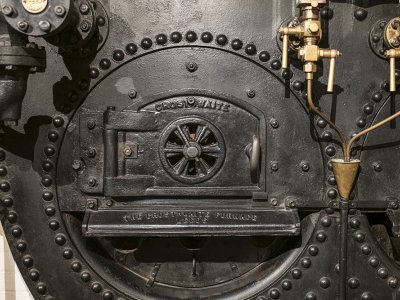The image depicts a detailed close-up of the front of an old-fashioned black iron furnace or boiler. The entire structure is made of black metal with a circular opening prominently featured, bordered by evenly spaced rivets. Inside this circular frame is a small dome-shaped door equipped with a six-spoke wheel in the center, a twistable vent, and a handle on the right side. Below the door, there is a protruding tray or ledge. The door is hinged on the left with heavy black iron hinges. Surrounding the circular opening and extending to the upper right corner are various brass fixtures, including knobs, handles, and copper tubing, possibly used for controlling steam or water flow. Though some writing is visible on the metal surface, it is not clearly legible. The apparent weight and antiquity of the machinery underscore its industrial heritage.